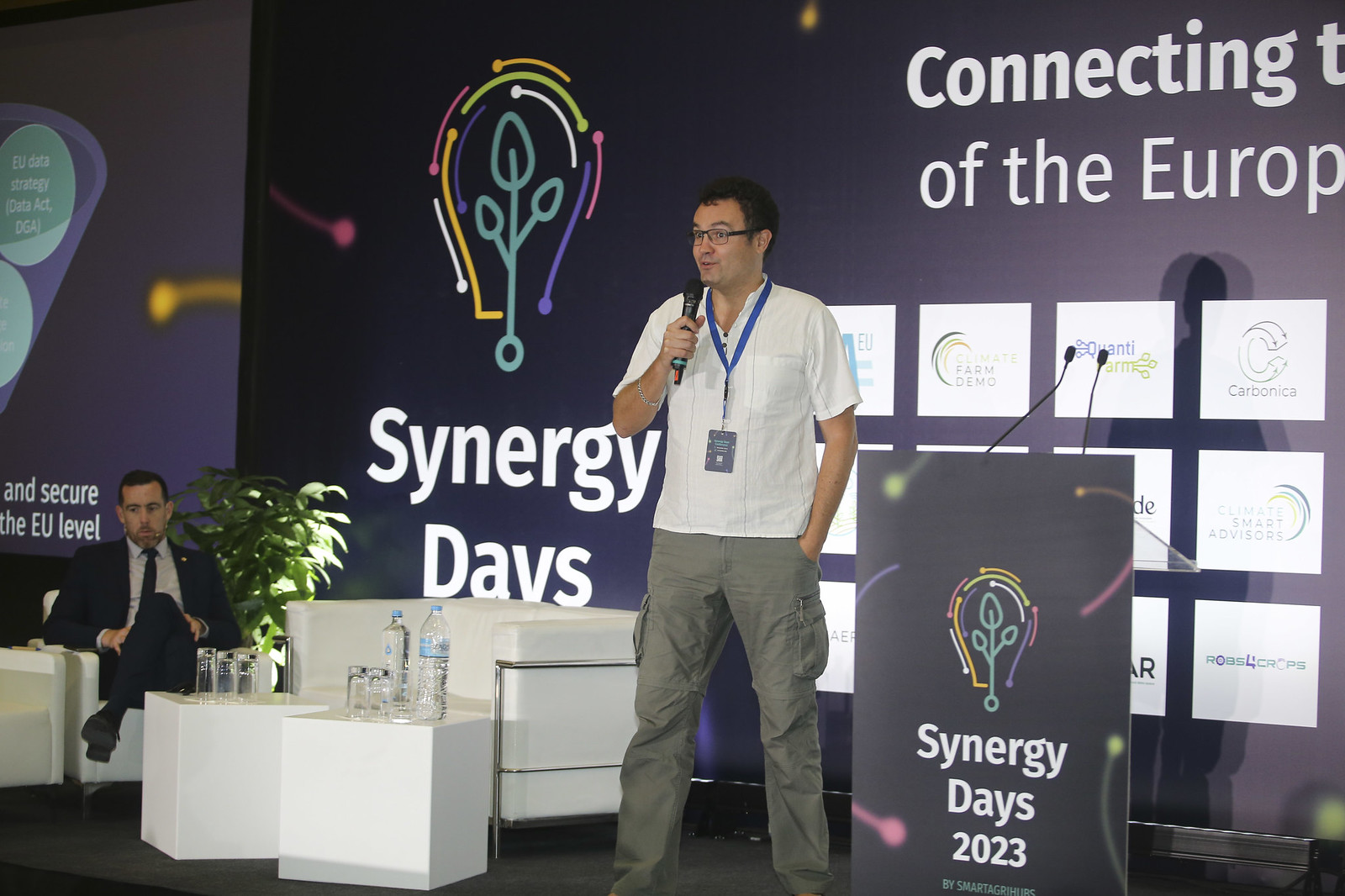In this detailed photograph of a corporate event titled "Synergy Days 2023," a man stands confidently on a stage, wearing a short-sleeve white t-shirt, gray cargo pants, and a lanyard. He has short black hair and is sporting dark-rimmed glasses. Holding a microphone close to his face with one hand while the other rests in his pocket, he addresses the audience, seemingly passionate about his topic.

To his left, a man dressed in a sharp suit is seated on a white chair amongst a few other unoccupied chairs and tables adorned with glasses and water bottles. On the right side of the speaker, there’s a podium featuring the event’s logo—a light bulb with a plant inside—and the text "Synergy Days 2023." Two smaller microphones extend from the top of the podium.

The background is dominated by a large screen displaying the same logo and branding words, "Synergy Days" and "Connecting in Europe" in white text against a dark backdrop with colors like green, white, purple, pink, and black. The setup and the ambiance suggest a well-organized forum or meeting focused on European connectivity and collaborative synergy.